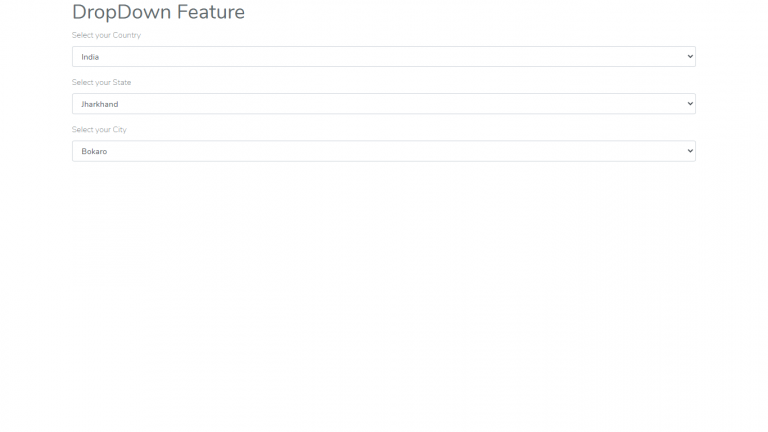In this image, we see a screenshot with text that is very light and somewhat difficult to read. The upper left corner features bold text that labels a drop-down menu. Below it, in even lighter text on the left side, instructions read "Select your category." This section includes a long drop-down box, which currently displays "India."

Beneath this, there is another set of instructions, "Select your state," accompanied by a second drop-down box displaying the text "Jharkhand."

Lastly, there is a third long drop-down box with the instruction "Select your city," which is currently set to "Bokaro."

The image itself is very simple, with a solid white background and three drop-down features labeled "Select your country," "Select your state," and "Select your city," respectively.